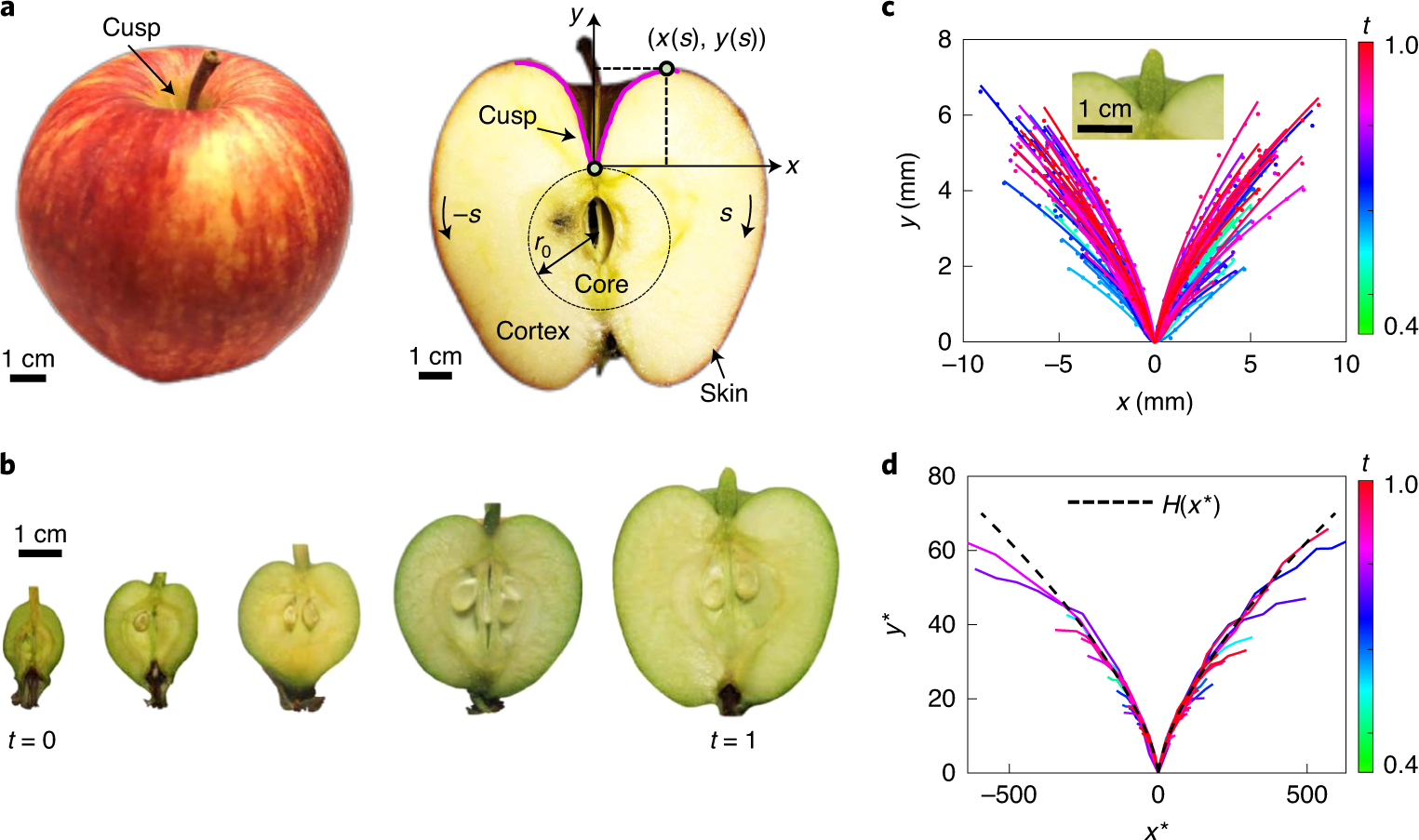The image is a scientific diagram displayed on a rectangular white background, where the top and bottom sides are significantly longer than the left and right sides. It features four distinct charts each labeled with a lowercase black letter. 

In the top left corner of the diagram, labeled with a lowercase black "A", there is a depiction of a red apple shown in two forms: whole and cut in half. The whole apple has a black arrow pointing to the stem area, labeled as "cusp". The halved apple is annotated with lines of black text pointing to various parts, including the divot at the top labeled "cusp", the central core circled and labeled "core", and the flesh of the apple labeled "cortex".

Below this, labeled "B", is a series of images illustrating the growth stages of a green apple, each stage showing the apple cut open to display the internal structure.

The top right section, labeled "C", contains a data plot. This plot is characterized by its V-shaped pattern with colors such as red, blue, turquoise, and purple radiating from the point where the x-axis intersects at zero. This graph appears to analyze some variable related to the apple's characteristics.

Directly below it, labeled "D", there is another graph with the x-axis ranging from -50 to 50 and the y-axis ranging from 0 to 80. This plot also has a V-shaped pattern centered at zero and includes mathematical notations like h(x), possibly representing another set of measurements or data related to the apple's properties.

Overall, the detailed annotations, data plots, and scientific labeling suggest that this image is a comprehensive scientific diagram examining various physical and mathematical aspects of an apple.